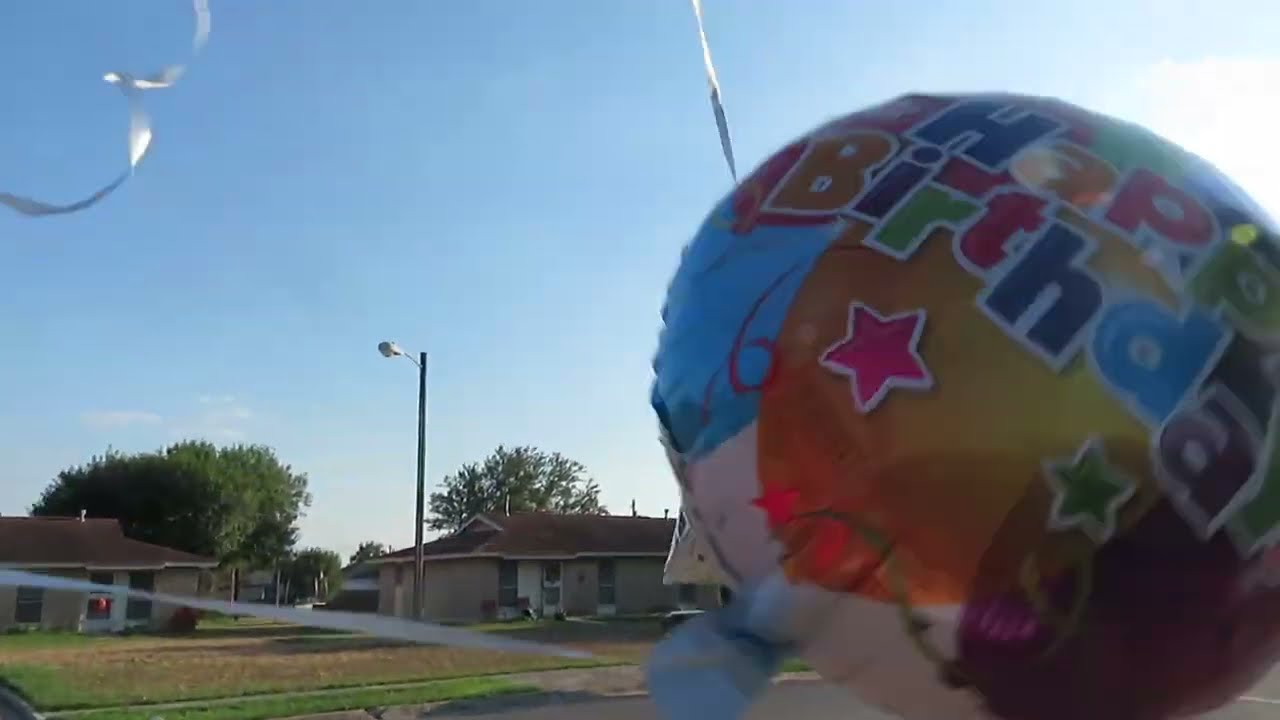In this vibrant outdoor image taken in a residential neighborhood during the day, the focal point is a shiny, metallic birthday balloon located in the bottom right corner. The balloon, slightly out of focus due to its proximity to the camera, features the text "Happy Birthday" with each letter in a different bright color. Below the text, the balloon is adorned with patterns of various colored balloons and stars, adding to its festive appearance. A white string tied to the bottom of the balloon stretches towards the left side of the image.

The scene extends to show a gray sidewalk lined with green grass, leading to two single-story houses that reside in the backdrop. These houses are characterized by white-framed windows and deep brown tiled roofs. The sky above is lightly clouded, adding depth to the setting. Additional elements in the image include trees, a streetlight, and well-kept lawns, enhancing the neighborhood's serene and charming atmosphere. The colors throughout the image include vibrant shades such as blue, red, orange, purple, green, pink, yellow, brown, and gray, creating a rich and detailed composition.